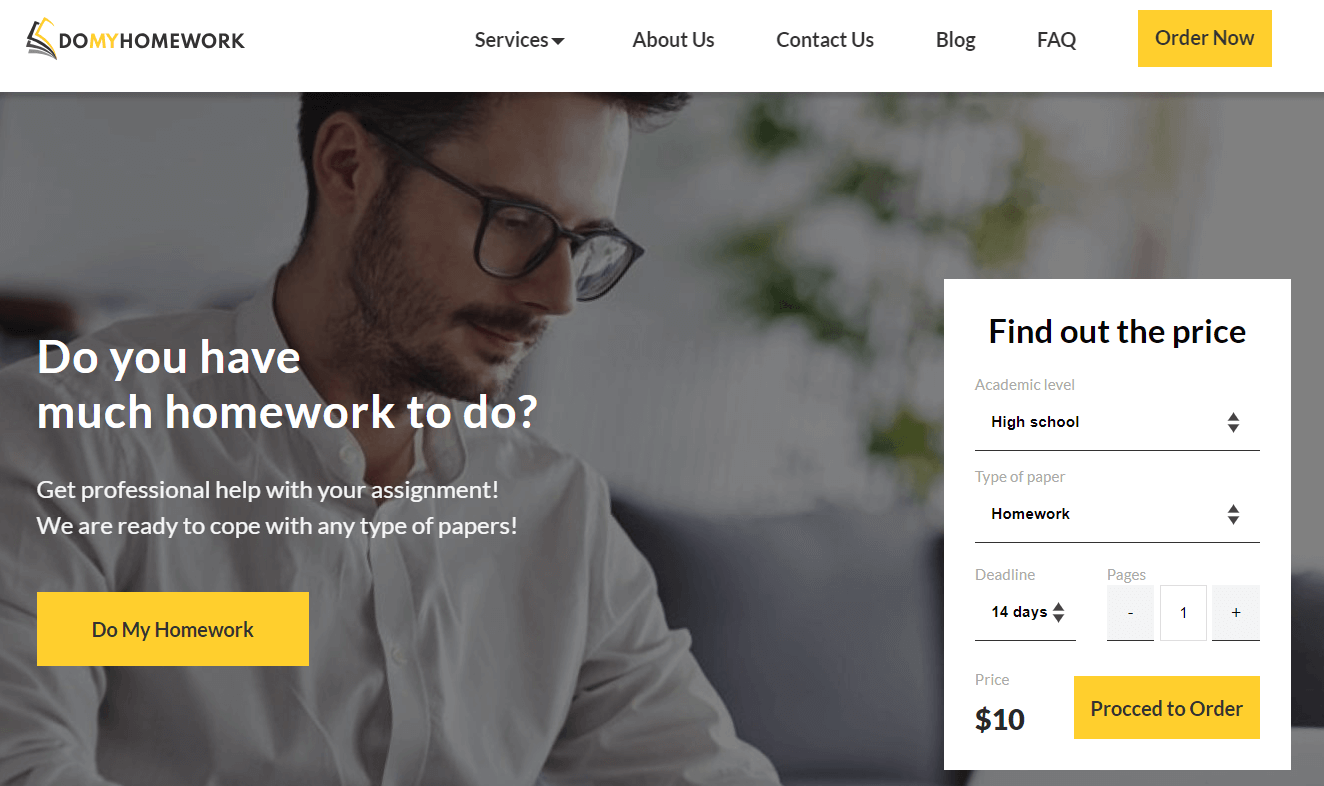The image is an order page for the website DoMyHomework (all one word), featuring a layout designed for potential clients seeking assignment assistance. 

On the left side of the page is the DoMyHomework logo, which resembles a stack of paperwork. The website navigation includes tabs for various sections such as Services (with a drop-down arrow), About Us, Contact Us, Blog, and FAQ. Prominently displayed is a bright yellow "Order Now" button.

The main image captures a young man, likely in his early 30s and of European descent. He has brown hair, a light beard, a mustache, and wears prescription glasses. Dressed in a white button-front shirt with a low collar, he appears to be looking down contemplatively.

The central text within a highlighted box inquires, "Do you have much homework to do?" and follows with a call to action: "Get professional help with your assignment! We are ready to cope with any type of papers!" A yellow button below the text prompts with "Do My Homework" (three separate words).

To the right of this text box is the "Find Out the Price" section. This white panel allows users to customize their order:

1. "Academic Level" – currently set to "Homework" with up and down arrows to adjust.
2. "Type of Paper" – also set to "Homework," with similar adjustment arrows.
3. "Deadline" – set at "14 days," adjustable with up and down arrows.

Below these fields are options for specifying the number of pages, formatted as vertical boxes with plus and minus options to add or subtract quantity. The calculated price is displayed as "$10," beneath which lies the "Proceed to Order" button for finalizing the request.